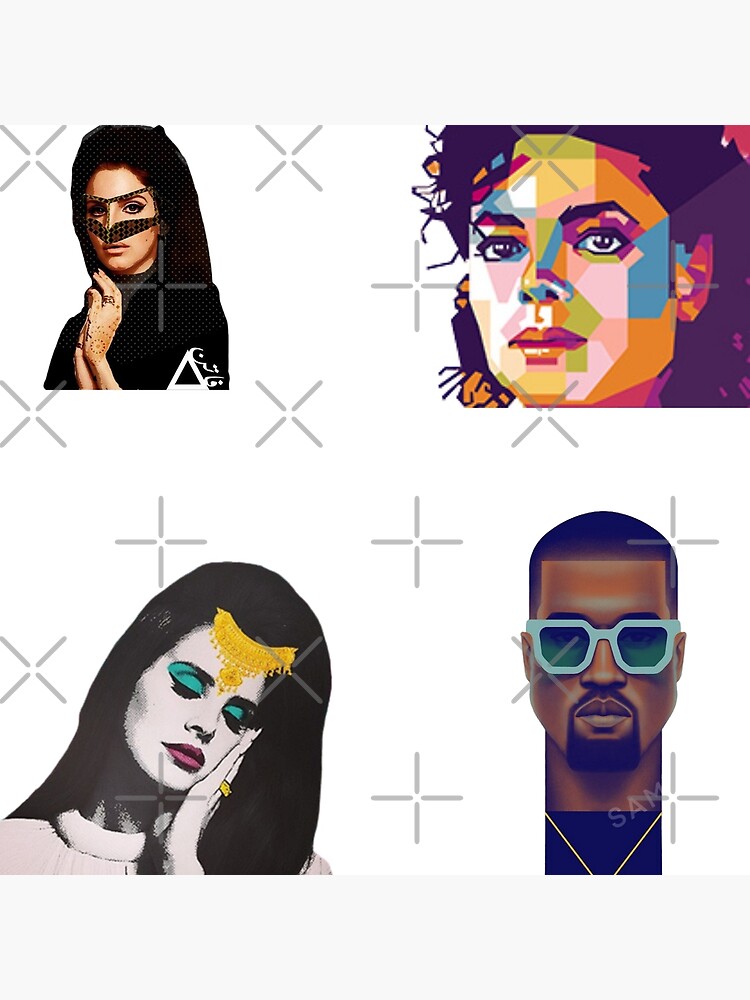This square-shaped image with a white background features a modern, digitally manipulated art piece with a beige bar on the top and bottom. At its center is a white square showcasing four celebrity faces, each created in a vibrant, computerized style reminiscent of Andy Warhol's pop art.

In the top right corner, Michael Jackson's pixelated visage is accentuated with geometric shapes and a myriad of colors—his forehead is yellow, side of his face blue, and varying sections splashed with pink, purple, and orange shades, giving his image a fragmented yet cohesive artistic look.

On the bottom right, Kanye West's face is rendered like a modern avatar, characterized by his dark skin, black goatee, black hair, and striking mint green glasses. He sports a black t-shirt and a gold chain, cementing his iconic style in a cartoon-like depiction.

The top left features a woman, possibly Amy Winehouse, with white skin and black hair. Her face is partially obscured with a mask-like filter, adding a unique texture. She has additional detailing like henna on her hand and an intriguing stacked triangle symbol by her arm reminiscent of Arabic designs.

Bottom left is another woman, likely Lana Del Rey. Her image is mostly black and white, with pronounced turquoise eyeshadow and red lipstick. She wears a gold tiara, blending the aesthetic of 70s and 80s pop art. Her figure also showcases bright makeup juxtaposed with a washed-out appearance, and she adorns a gold headpiece and a gold ring.

Throughout the image, there are plus and X symbols that resemble watermarks, further enhancing its modern, stylized look.